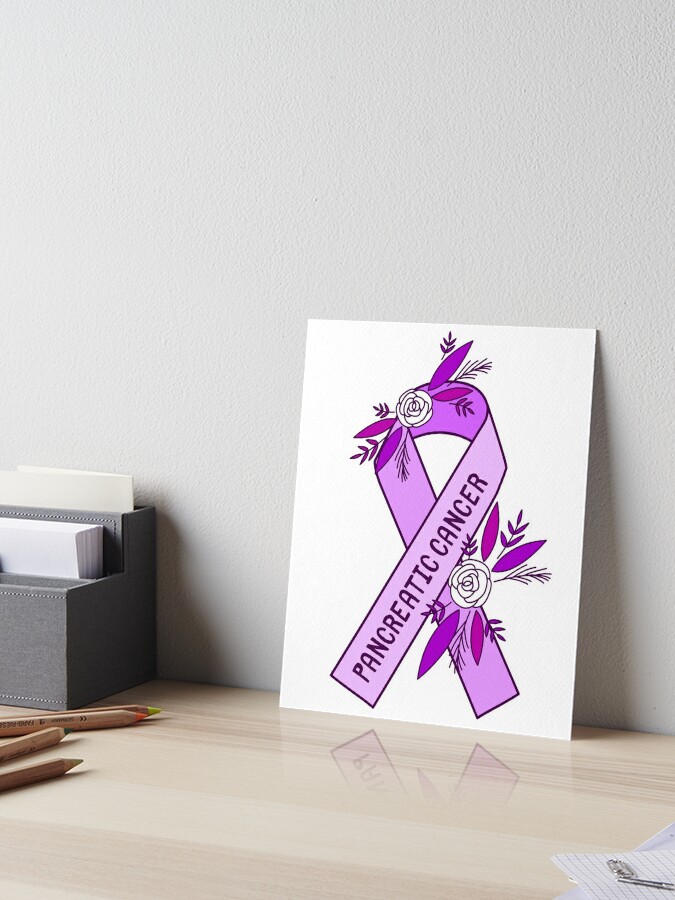The photorealistic image depicts a wooden desk with a reflective glass surface, against a white or grey wall. Leaning against the wall is a postcard or poster primarily featuring a prominent purple ribbon with the text "pancreatic cancer". The ribbon is adorned with white roses at both ends, detailed with purplish leaves and stems. To the left of the postcard, there is a black, piano-shaped stationery organizer containing various papers. In front of the organizer lies a set of four colored pencils—yellow, orange, green, and another yellow—each with wooden bodies and colored tips. Additionally, scattered on the lower right corner of the desk are pieces of paper with paper clips on top. In the background, partially visible, is some sort of cabinet likely used to hold folders, along with small wooden spears scattered on the floor. The overall setting suggests a work or study space with a focus on pancreatic cancer awareness.